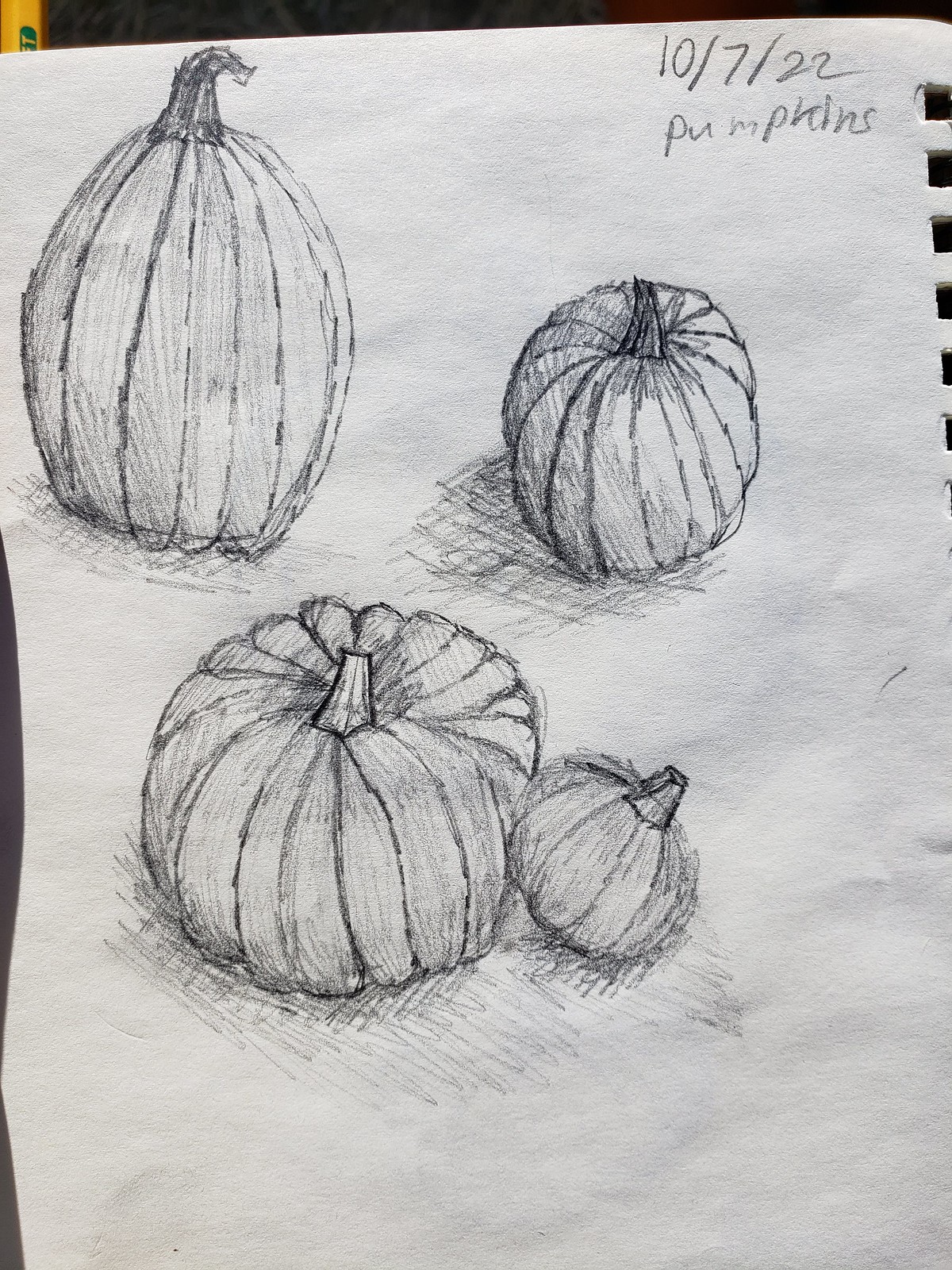In this detailed pencil sketch, four distinctively drawn pumpkins are depicted against a black background, emphasizing the contrast with the white piece of paper. The sketch appears to be on a notepad, evidenced by the torn spiral notebook edge on the far right and the small perforated boxes visible. At the top right, the date "10/7/22" is inscribed, with the word "pumpkins" written beneath it in handwriting. 

Central to the composition is a large, wider, and shorter pumpkin with a tiny pumpkin leaning against it at a 45-degree angle. To the upper left, there's a taller, skinnier pumpkin with a curved stem pointing to the right, while the upper right features a smaller, circular pumpkin. To the right of the central pumpkin, a bowl-shaped pumpkin completes the arrangement. Each pumpkin is meticulously shaded with crisscross pencil strokes, giving them a scratchy texture, and detailed with darker stems. The shading underneath each pumpkin creates the illusion of them either resting on a surface or casting shadows, adding depth to the sketch.